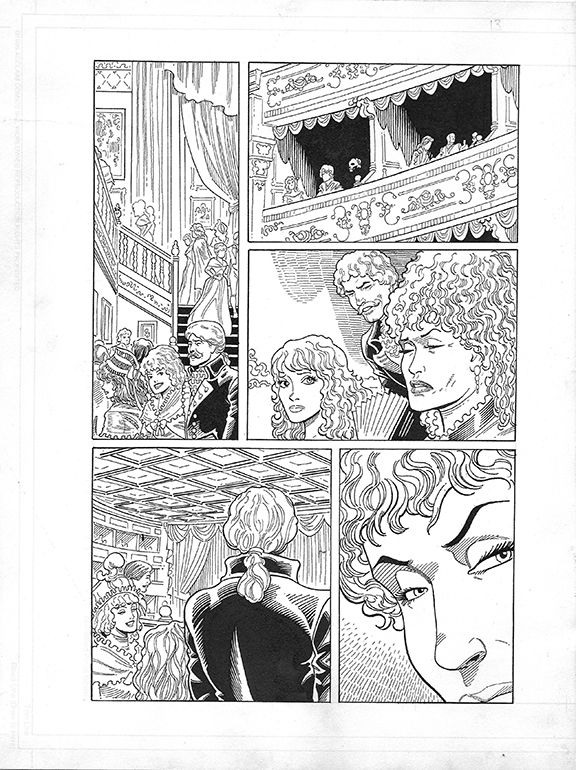This detailed black and white pencil drawing is a comic book page, styled like an old magazine, featuring intricate and highly stylized artwork across five panels. The top left panel, a tall rectangle occupying two-thirds of the page vertically, depicts a lavish gathering in an opulent, historic theatre or mansion, complete with artwork-adorned walls and grand double winding staircases. The elegantly dressed attendees, donned in ruffled suits and elaborate outfits, appear to be descending the staircase. The adjacent top right panel showcases some of these guests seated in a fancy balcony area, resembling royal boxes, intently watching a stage performance with curtains partially visible in the background.

Moving down, the third panel captures a tense moment between three characters. Two women with elaborate curly hair appear displeased, while a mischievous-looking man, possibly the source of their ire, stands nearby. Below this, the bottom left panel offers a rear view of this cheeky man, characterized by his ponytail, as he gazes towards the stage, surrounded by further elegantly attired spectators beneath a decorative ceiling.

The bottom right and final panel zooms in on one of the aforementioned women, her eyebrows raised in suspicion or concern as she directs her gaze off to the side, away from the viewer’s perspective, hinting at an unfolding drama or intrigue within this richly detailed and atmospheric scene.